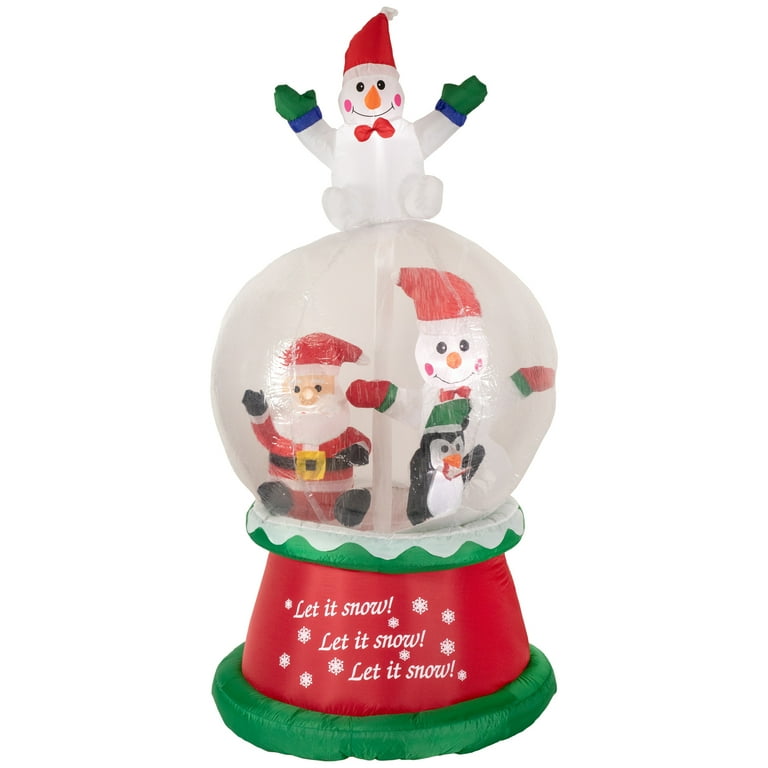The image features a festive Christmas snow globe prominently displayed against a white background. The base of the snow globe is a green circular platform adorned with a red structure that bears the phrase "Let it snow, let it snow, let it snow" in white text and white decorative designs. Inside the clear, dome-like enclosure of the snow globe, a vivid scene comes to life with animated figures of Santa Claus, a snowman, and a penguin. Santa Claus is dressed in his traditional red and white outfit. The penguin sports a green Christmas hat, and the snowman is outfitted with a red Christmas cap, red and orange gloves, and a red bow tie. Atop the globe, another white snowman, accentuated with a red hat, green and blue gloves, and a red bow tie, sits proudly. The colors throughout the scene include greens, whites, reds, blacks, gold, orange, and blue, enhancing the overall festive atmosphere of this Christmas-themed decoration.